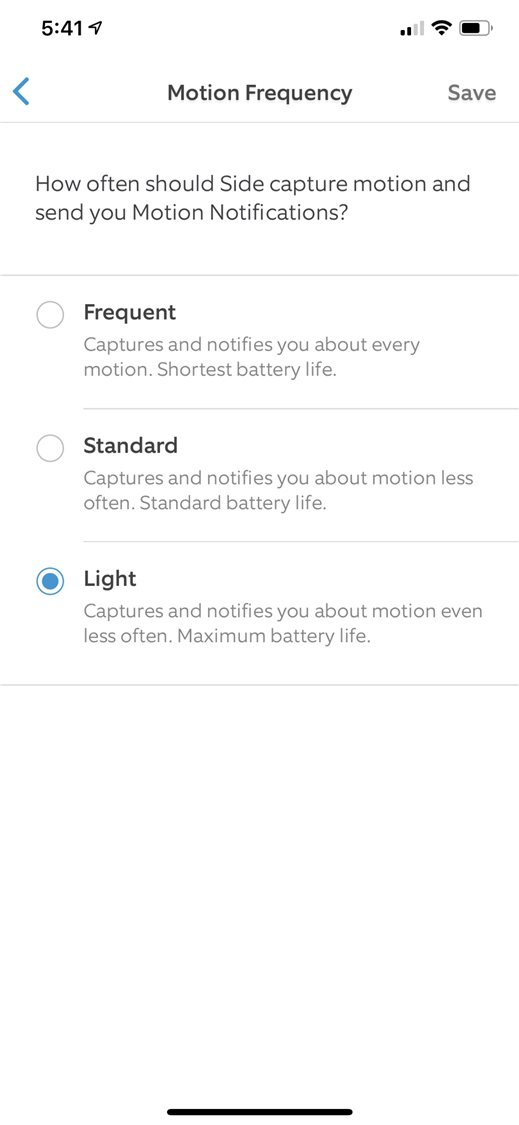A screenshot from a smartphone, showing the "Motion Frequency" settings menu. The time displayed is 5:41, and the device has a low signal strength but a high battery charge. The screen title "Motion Frequency" indicates the current setting, guiding the user on how frequently motion is detected and notifications are sent. Three options are available: 

1. **Frequent**: Captures and notifies about every motion, resulting in the shortest battery life.
2. **Standard**: Captures and notifies about motion less often, providing standard battery life.
3. **Light** (currently selected): Captures and notifies about motion even less often, ensuring maximum battery life.

The menu emphasizes the trade-off between notification frequency and battery consumption, without offering the option to disable motion detection entirely. This suggests that motion detection is a crucial feature of the device.